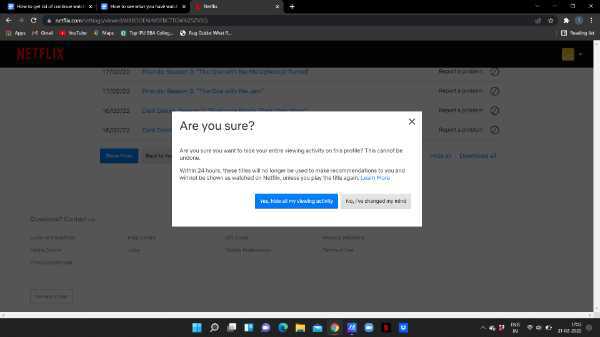The image depicts a computer screen displaying a web page, specifically the Netflix site, recognizable by the prominent red Netflix logo in the upper left corner. The website appears to be grayed out, indicating a pop-up message in the foreground. The pop-up features a white box with the question "Are you sure?" accompanied by two clickable options: a blue "No" button and a gray "Yes" button to the right.

The user has three browser tabs open, with the Netflix tab being the current one in focus. Two other tabs are visible to the left of the current tab. At the bottom right corner of the screen, the time is displayed as 11:17, alongside various system icons positioned at the bottom center of the screen. The top toolbar is densely populated with numerous app icons for quick access.

The overall color scheme of the image includes shades of gray, black, red, and blue, contributing to a minimalist yet functional interface.